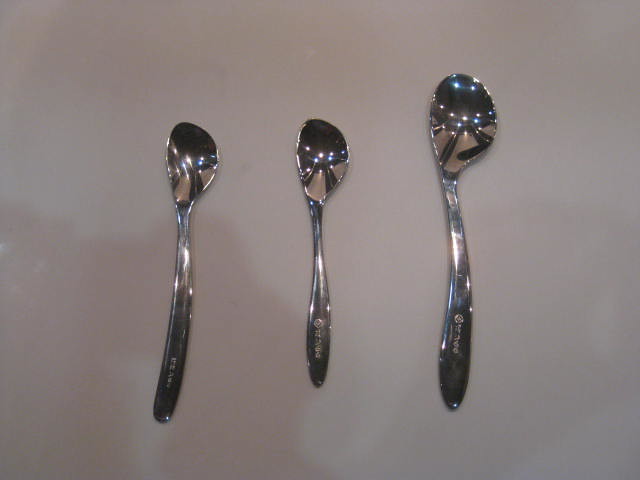The photograph captures three shiny, slightly varying-sized spoons lying on a beige background, arranged from the bottom left to the top right in a staggered, step-like fashion. Each spoon is positioned bowl-side down, revealing their highly reflective, polished surfaces that capture and reflect bright orange and bluish lights. Shadows cast predominantly in the lower left corner of the image suggest an overhead lighting source. While the spoons are not evenly spaced, the largest spoon situated to the right resembles a serving spoon, the smallest in the middle appears to be a teaspoon, and the medium-sized spoon on the left is akin to a soup spoon. All three handles display an engraved logo and some letters or numbers, although the specific details are not legible. The handles also show a progression towards a more shaded or tarnished appearance near their ends.